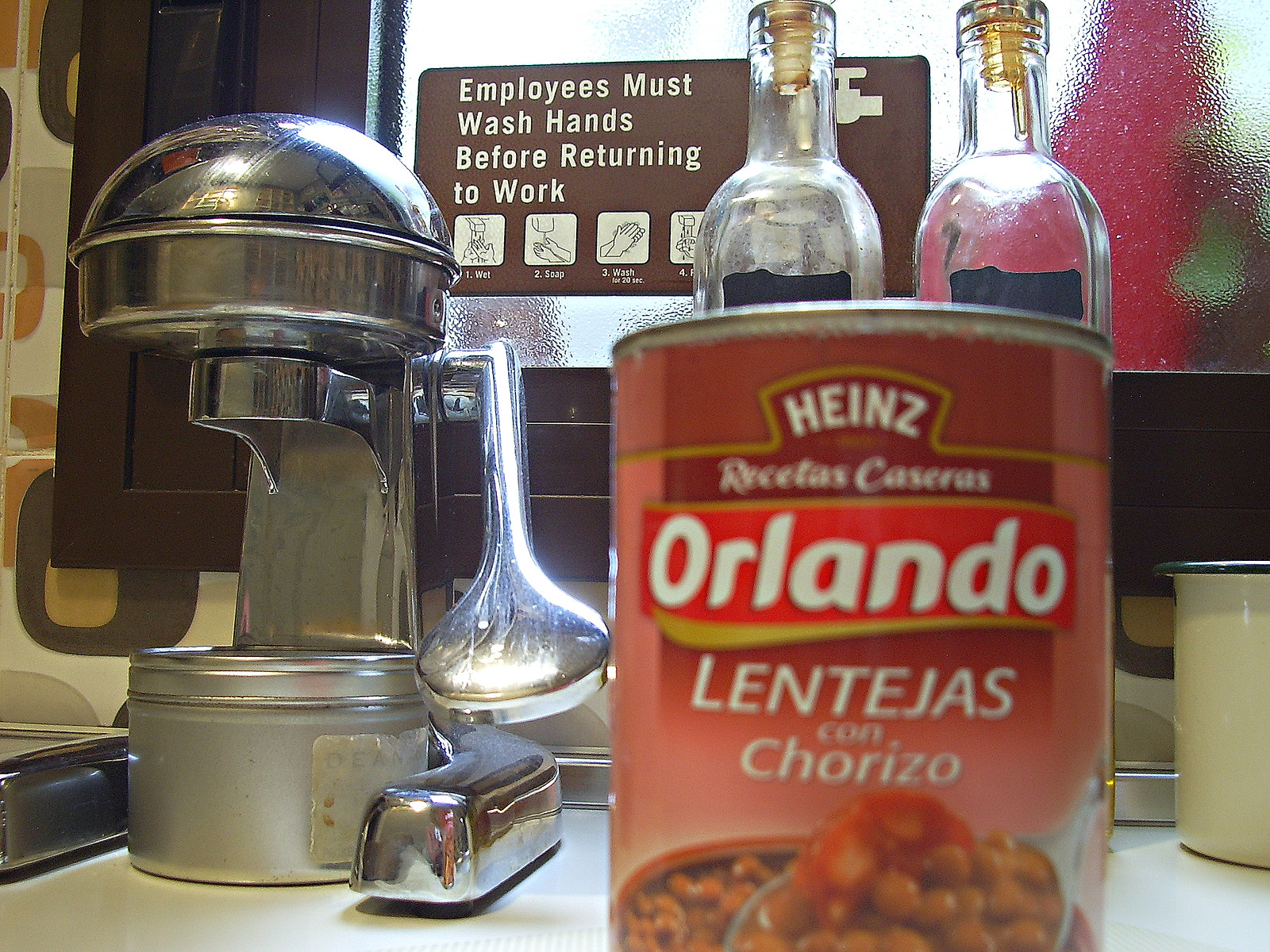The image captures a close-up scene of a restaurant counter. On the counter, various food items are present, confirming the setting as a restaurant. Behind the counter, a frosted window glass features a small sign that reads, "Employees must wash hands before returning to work," accompanied by illustrated steps on proper handwashing techniques. Prominently displayed at the front is a can of Heinz Orlando Lentejas con Chorizo, featuring an image of lentils or beans on its label. Additionally, there is a large silver device resembling a citrus squeezer, complete with a substantial handle and an apparatus designed to press fruit. The base of this squeezer includes a platform where a glass can be placed to collect the freshly squeezed juice.